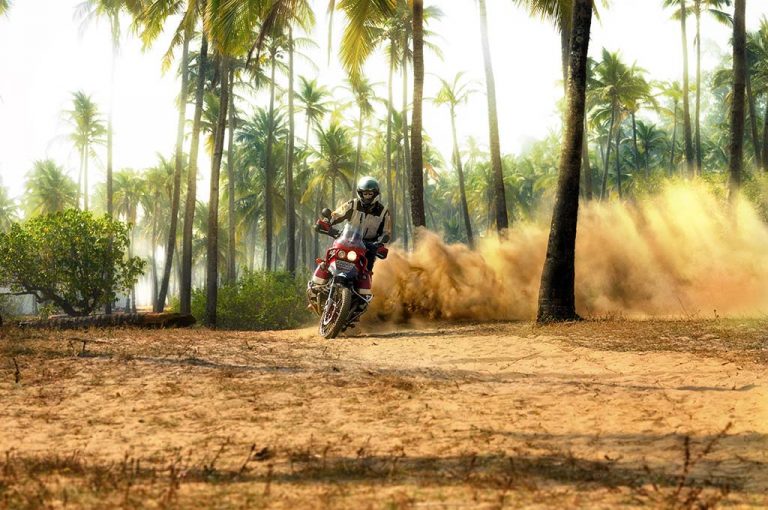In the image, a person is captured riding a red and white motorcycle through a sandy, dirt-laden area that could be near a beach due to the presence of sandy soil mixed with patches of sparse grass and weeds. The scene is set outdoors under a partly cloudy sky, featuring hues of white and light blue. The background is populated with tall, green palm trees, suggesting a tropical environment, with palm leaves and trunks visible, and rays of light filtering through. 

The motorcyclist, potentially a man based on the attire, is dressed in a protective outfit, including a black and white jacket and a dark, possibly green helmet, indicative of the careful attire required for off-road conditions. The single headlight on the red motorcycle is visible, and the rider appears to be steering slightly to the right, generating a noticeable plume of dust and smoky exhaust, indicating motion and speed.

In this detailed portrayal, the earthy tones of brown and yellow sand contrast with the lush greenery of the palms, establishing a vibrant yet rugged atmosphere unique to this outdoor setting. The left side of the image features a prominent trunk, and a downed log lies nearby, further enhancing the sense of a natural, untamed landscape.